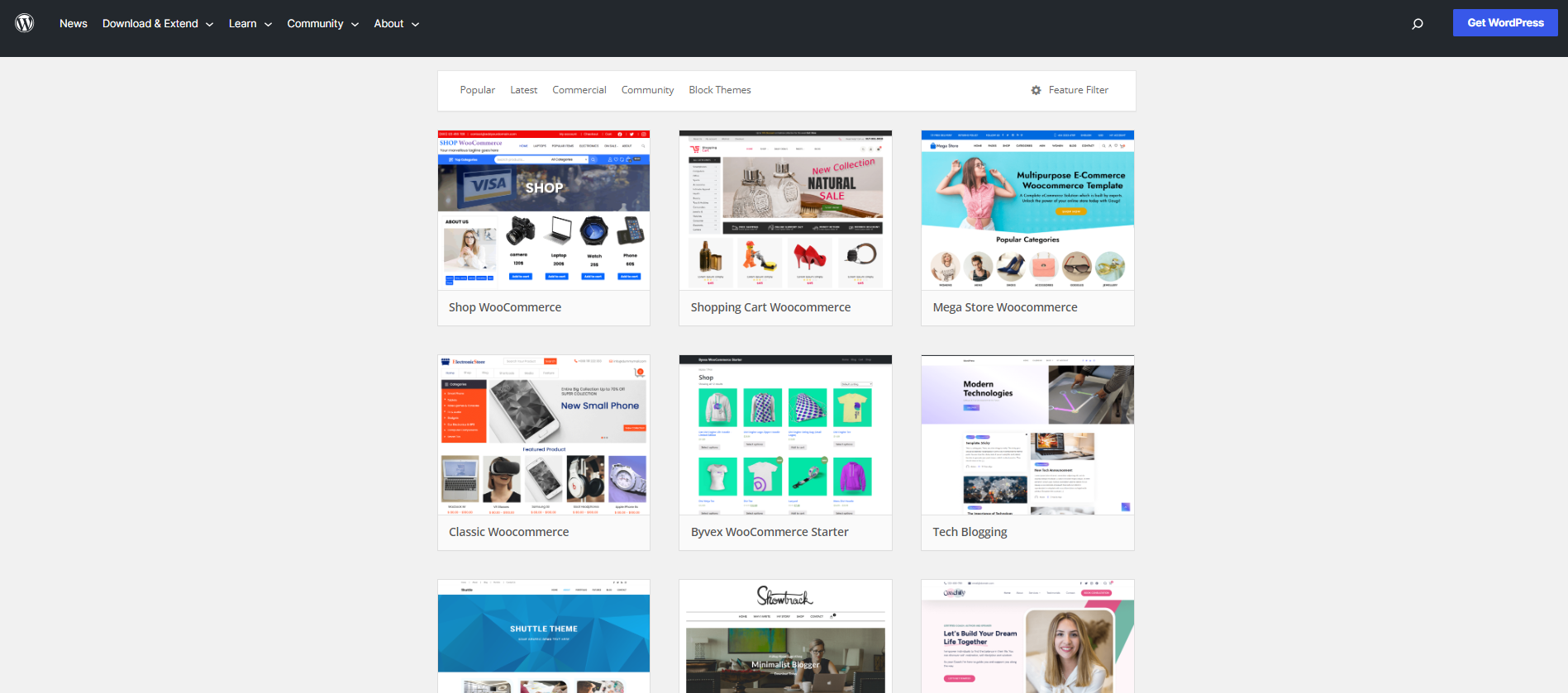This screenshot captures a WordPress theme browsing page. In the top left corner, the WordPress logo is prominently displayed, along with navigation options labeled News, Download & Extend, Learn, Community, and About. In the top right corner, a blue button marked "Get WordPress" stands out. Just below is a horizontal white banner offering a variety of options: Popular, Latest, Commercial, Community, and Block Themes. To its right, a "Feature Filter" option is available.

Occupying the main section below the banner are images representing nine different webpage themes. The first image, titled "Shop WooCommerce," showcases a shopping site displaying various products. Adjacent to it, "Shopping Cart WooCommerce" also features product images, including a noticeable pair of Red High Heels. "Megastore WooCommerce," the next image, displays people donning various clothing items, along with pictures of a pink purse and sunglasses.

Beneath these, "Classic WooCommerce" presents a landing page with a featured image of a cell phone, followed by products such as a watch and a laptop. Next to it, "Byvex WooCommerce Starter" is depicted with a white page background and green product boxes. On the far right, "Tech Blogging" is displayed.

The final row shows three more themes, though their bottom parts are cut off. "Shuttle Theme" is the first one, while the middle one appears to read "Show Track" or "Show Brack" in cursive script. The last screenshot features a headline proclaiming, "Let's Build Your Dream Life Together."